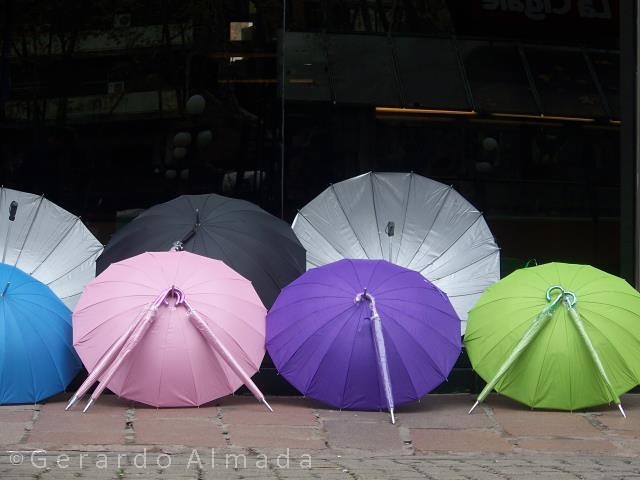This photograph captures a darkened storefront serving as a backdrop for a striking display of colorful umbrellas laid out on a cobblestone sidewalk. The background features old, possibly unused, electrical fixtures, giving a vintage feel to the scene. The storefront window is black and reflective, further accentuating the vibrancy of the umbrellas in front. 

On the sidewalk, there are two distinct rows of open umbrellas. The back row, from left to right, features a partially visible inside-out silver umbrella, followed by a fully open black umbrella, and another open silver umbrella viewed from the inside. In front of these, a row of open umbrellas showcases a diverse palette: a pale blue umbrella on the far left, followed by a light pink umbrella with three closed pink ones hooked onto it, a purple umbrella with a single closed purple one attached, and a green umbrella with two closed lime green ones hanging from it. 

There is text watermarked in the lower left corner of the image, which reads "Gerardo Almada."